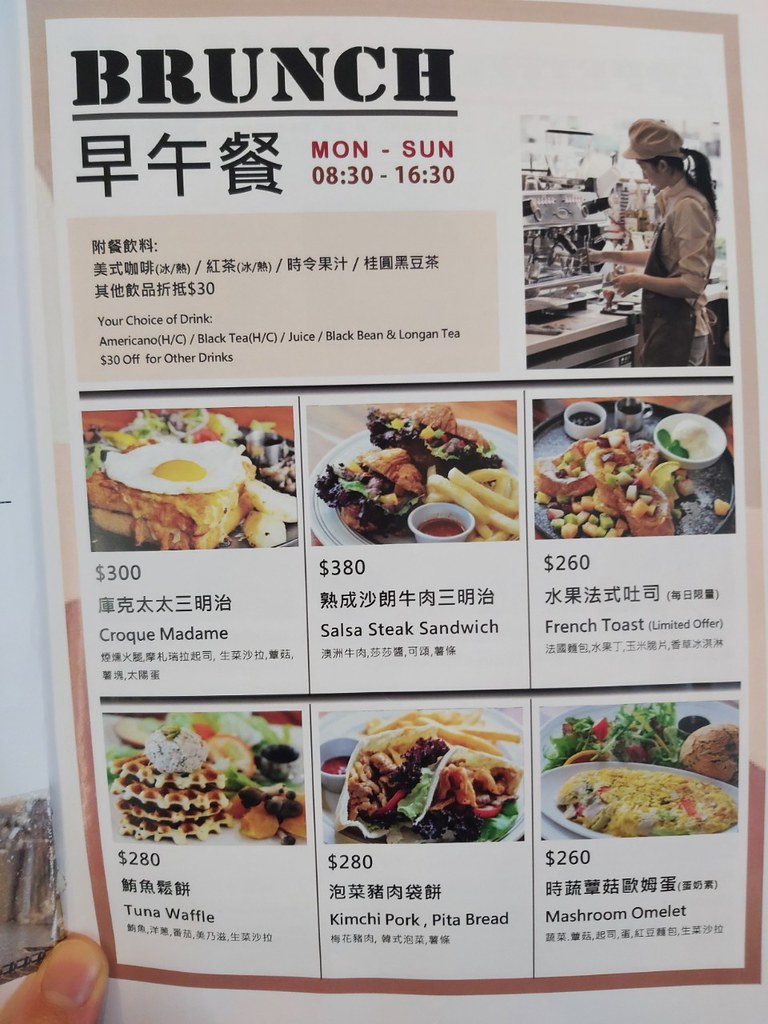The image features a bilingual brunch menu with both Asian language text and English. The word "BRUNCH" is prominently displayed at the top in bold, black capital letters. The establishment operates daily from Monday to Sunday, 8:30 AM to 4:30 PM. The beverage options listed include Americano (H/C), black tea (H/C), juice, black bean tea, and longan tea, with a 30% discount on alternative drinks.

In the top right corner, there is a photograph of an Asian female, possibly a chef, barista, or server, standing behind a counter. The menu showcases six distinct brunch items, each accompanied by a photo and price:

1. **Croque Madame** - priced at 300
2. **Salsa Steak Sandwich** - priced at 380
3. **French Toast** - priced at 260 (noted as a limited offer)
4. **Tuna Waffle** - priced at 280
5. **Kimchi Pork in Pita Bread** - priced at 280
6. **Mushroom Omelet** - priced at 260

A light-skinned individual is holding the menu, with just their thumb and a portion of their finger, including the thumbnail, visible in the image.